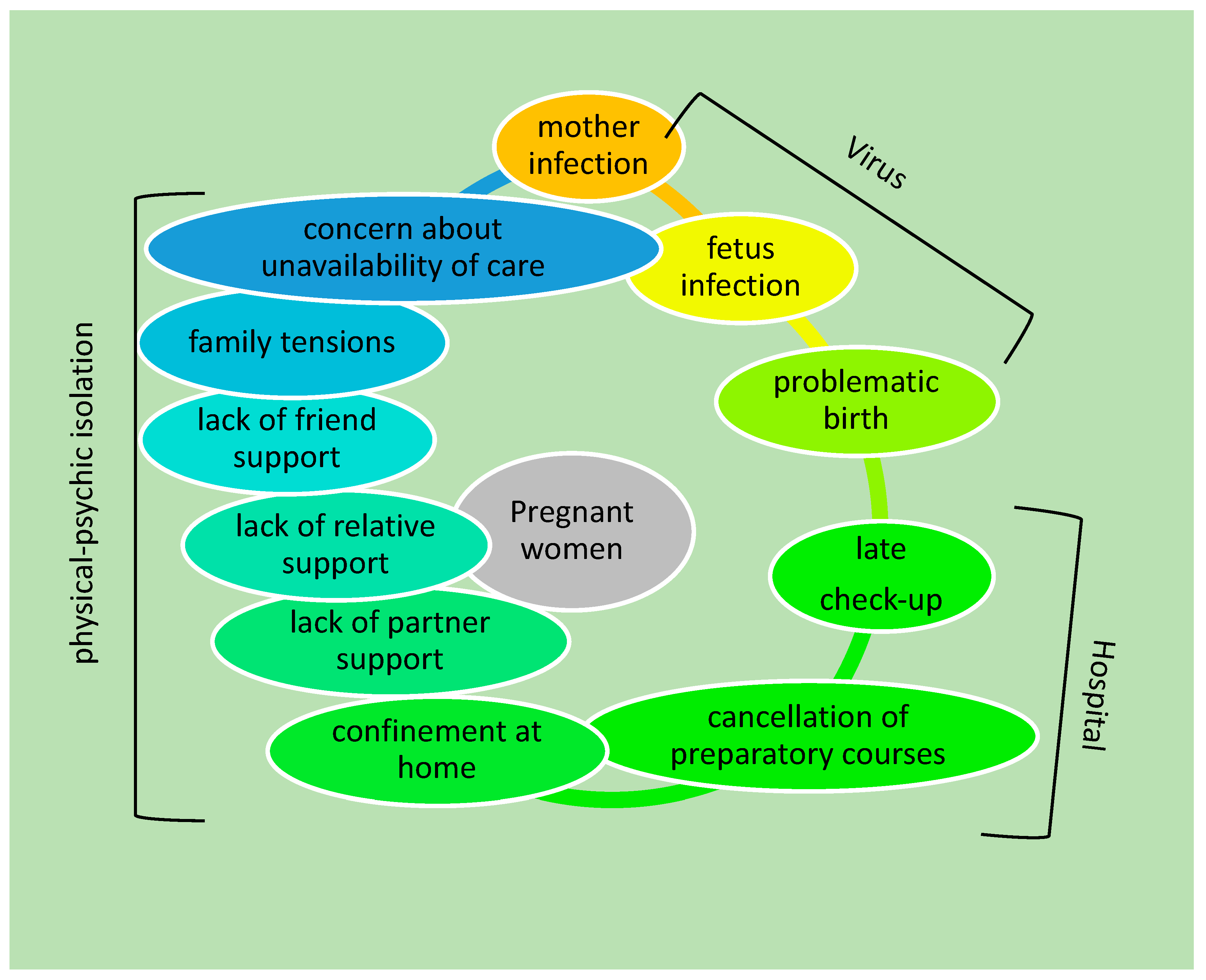The infographic is a circular flowchart titled "Physical and Psychic Isolation," designed to depict challenges faced by pregnant women. The illustration is set against a bright neon green background and is divided into three main sections: "Virus," "Hospital," and "Physical & Psychic Isolation," each color-coded with various text bubbles. 

Starting in the "Virus" section at the top right, it addresses issues such as mother infection, which can lead to fetus infection, and subsequently, problematic birth. This transitions into the "Hospital" section detailing late checkups and the cancellation of preparatory courses. The flow then moves into the "Physical & Psychic Isolation" section, outlining confinement at home, lack of support from partners, relatives, and friends, family tensions, and concerns about inadequate care availability. These challenges loop back to a mother infection, forming a continuous cycle. At the center of this cycle is a note highlighting its relevance to pregnant women. The graphic uses rudimentary, early PowerPoint-style visuals with poorly shaped ovals, which, despite their simplicity, underscore the severity and interconnectedness of the issues presented.